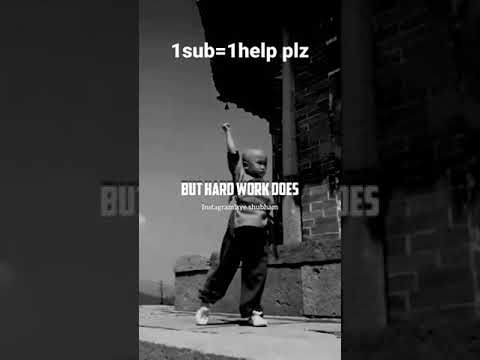The image is a black and white photograph featuring a young boy, approximately five or six years old, walking along a sidewalk next to a brick building. The boy is bald and is seen triumphantly raising his right arm in the air, creating a sense of determination. He is dressed in a light-colored shirt, long dark pants, and light-colored shoes. The background features an expansive sky, though it is unclear if it is overcast or sunny due to the monochrome effect.

Overlaying the image, there is bold white text. Near the top of the image, it reads: "one sub equals one help PLZ." Across the boy’s chest, in all capital letters, it says: "BUT HARD WORK DOES." Beneath this, there is a line of text that is too small and blurry to read. The photograph is framed by thick, gray borders on either side, which appear to be enlarged and grayed-out sections of the original image, creating a distinctive border around the central, impactful scene.